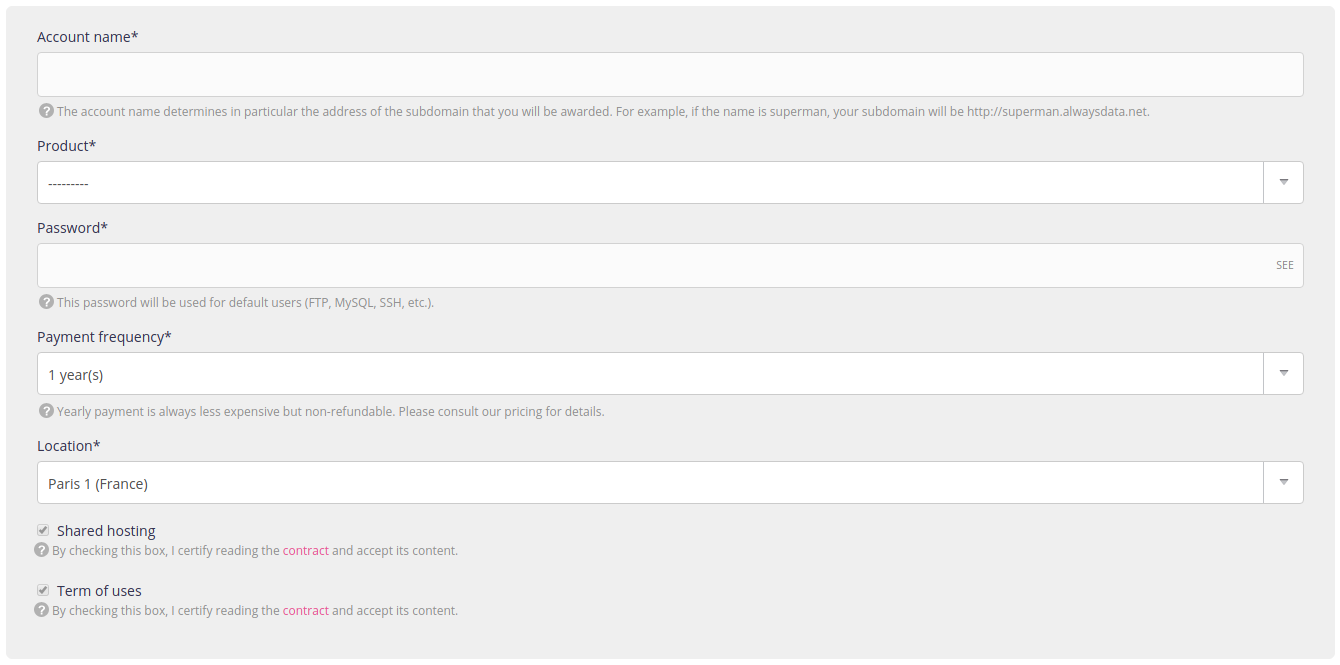Screenshot of a Gray Online Form Interface

The image is a wide, gray-background screenshot of an online form featuring several fields for user input. At the very top, the label "Account Name" instructs users that the entered name will determine their subdomain's address on the platform, giving the example "http://superman.alwaysdata.net" for clarity. Below this, the "Account Password" field is designated for creating a password that will be used for various system services including FTP, MySQL, and SSH.

Further down, the "Payment Frequency" field indicates a selection of a one-year payment term, noting that yearly payments are less expensive but non-refundable, with a prompt to consult the pricing details. The "Location" field is filled with "Paris 1, France."

The "Shared Hosting" option is checked, signifying the selection of a shared hosting plan. Two boxes labeled "Terms of Use" are also checked, certifying that the user has read and accepted the contract's content. The word "contract" is highlighted in red, indicating it is a clickable hyperlink.

The form has no photographic elements, humans, animals, plants, flowers, trees, or buildings. It is purely a form layout, intended for the setup and configuration of a web hosting account.